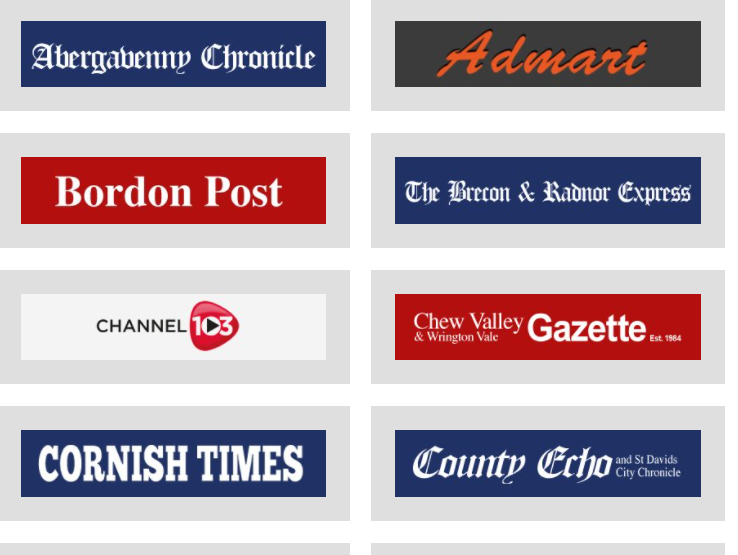This image features a website listing various local newspapers arranged in a grid format with a clean, white background. The dimensions of the image suggest a portrait orientation with a height to width ratio of approximately 55:45. The layout consists of two columns with four items each, making a total of eight listings. Each newspaper is represented by a long, gray horizontal rectangle paired with a smaller, colored horizontal rectangle, all bordered in gray and containing the titles and fonts specific to each paper.

From left to right and top to bottom, the newspapers are as follows:

1. "Abergabene Chronicle" - Displayed in a blue box with a font resembling Times New Roman.
2. "AdMart" - Featured in italicized orange and black.
3. "Borden Post" - Presented in white font within a red box.
4. "Brecon and Radnor Express" - Illustrated in a gothic style script in a blue box.
5. "Channel 103" - The number 103 is on a rectangle with rounded edges against a white background.
6. "Chew Valley and Rington Vale Gazette" - The title appears with an 'Estimate 1984' mark in a red box.
7. "Cornish Times" - The title is in all caps within a blue box.
8. "Country Echo" and "St. David’s City Chronicle" - Both titles are depicted in a blue box.

The design elements and fonts are tailored to reflect the identity and character of each newspaper, providing a clear and organized display of local media options.